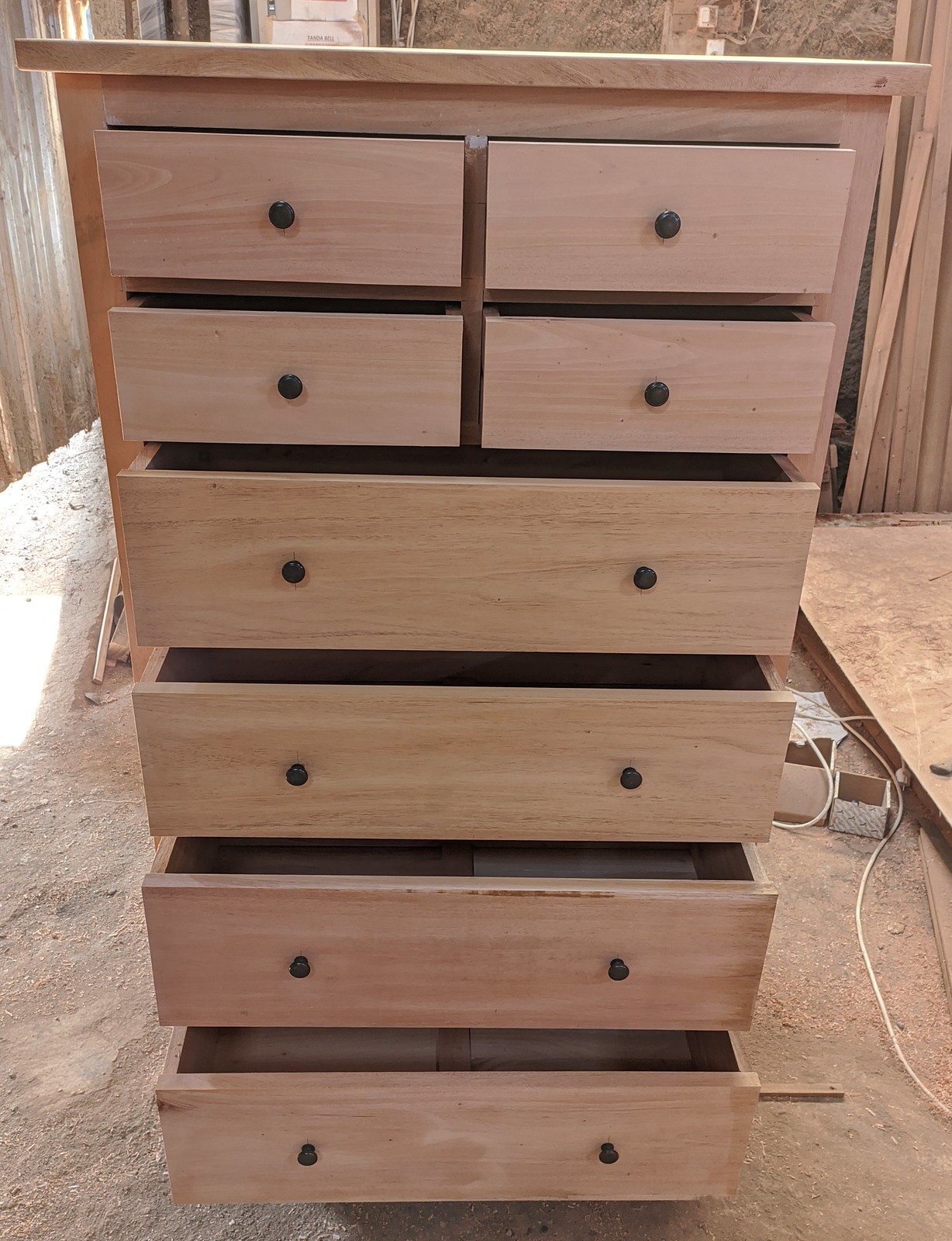The image depicts a tall, unfinished wooden chest of drawers situated in a workshop or construction site. It consists of four full-length drawers at the bottom, all partially open in a staggered manner, and four half-length drawers along the top. The knobs on the drawers are black, with two knobs on each of the full-length drawers and one knob on each of the half-length drawers, all aligned in a straight line. The background features an industrial setting with bare, exposed particle board walls, dirt and sawdust on the ground, along with scattered small cardboard boxes and white cords. Sunlight streams in from the left, adding a hint of the outdoor surroundings to the scene. Overall, the chest of drawers, made of light-colored wood, appears to be in its construction phase.